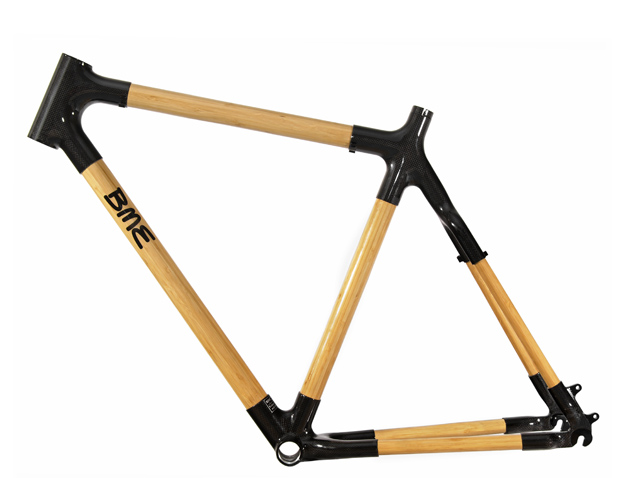The image features a geometric structure that resembles a bicycle frame. The primary shape is a polygon with four outer sides and one inward-angled side. This inward-angled side divides the polygon into two smaller triangular segments. Each of the polygon's corners is reinforced with black braces, which appear to be pre-fabricated for added stability. The connecting segments seem to be made of a light-colored wood, though the exact material is difficult to ascertain. The structure also features a small engraving of the letters "BME" on one of its parts, adding a distinctive mark to the design.